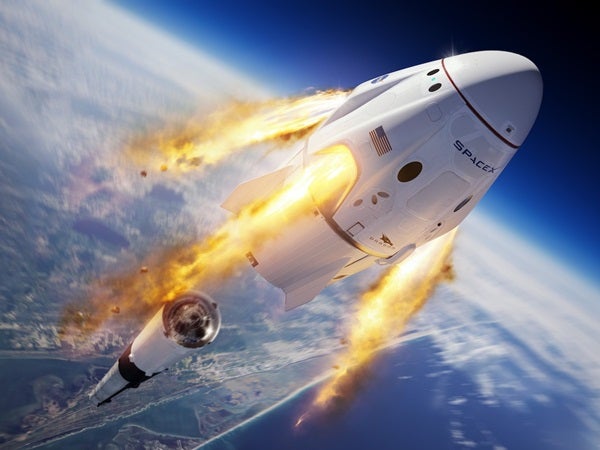In this dramatic image captured from space, the scene showcases the SpaceX Dragon capsule during a crucial moment—likely an emergency abort sequence. The capsule, prominently positioned in the foreground, is depicted launching away from a lower rocket stage, which trails behind it to the left. The Dragon capsule features a smooth, rounded white top with a thin black line encircling it, followed by a larger white body that bears a distinctive flag and the bold “SpaceX” in black lettering near the top section. 

Visible at the base of the capsule are the escape engines, emitting fierce flames that angle slightly left and down, indicating the forced separation from the rocket stages below. These flames are especially pronounced from three ports visible on the Dragon capsule, with likely a fourth hidden from view. This fiery propulsion marks the capsule's urgent maneuver away from the main rocket body.

The backdrop intensifies the scene, revealing the majestic curvature of Earth. The bottom two-thirds of the image displays a cloud-covered expanse, with hints of ocean and landmass, possibly the coastline of Florida. Above this terrestrial vista, the atmosphere transitions beautifully from a vivid blue near the horizon to the inky black of space in the upper third of the frame.

The image powerfully captures this tense moment of separation, with the Dragon capsule thrusting away from the distant rocket stage, accentuating the technical prowess and high stakes of space travel.